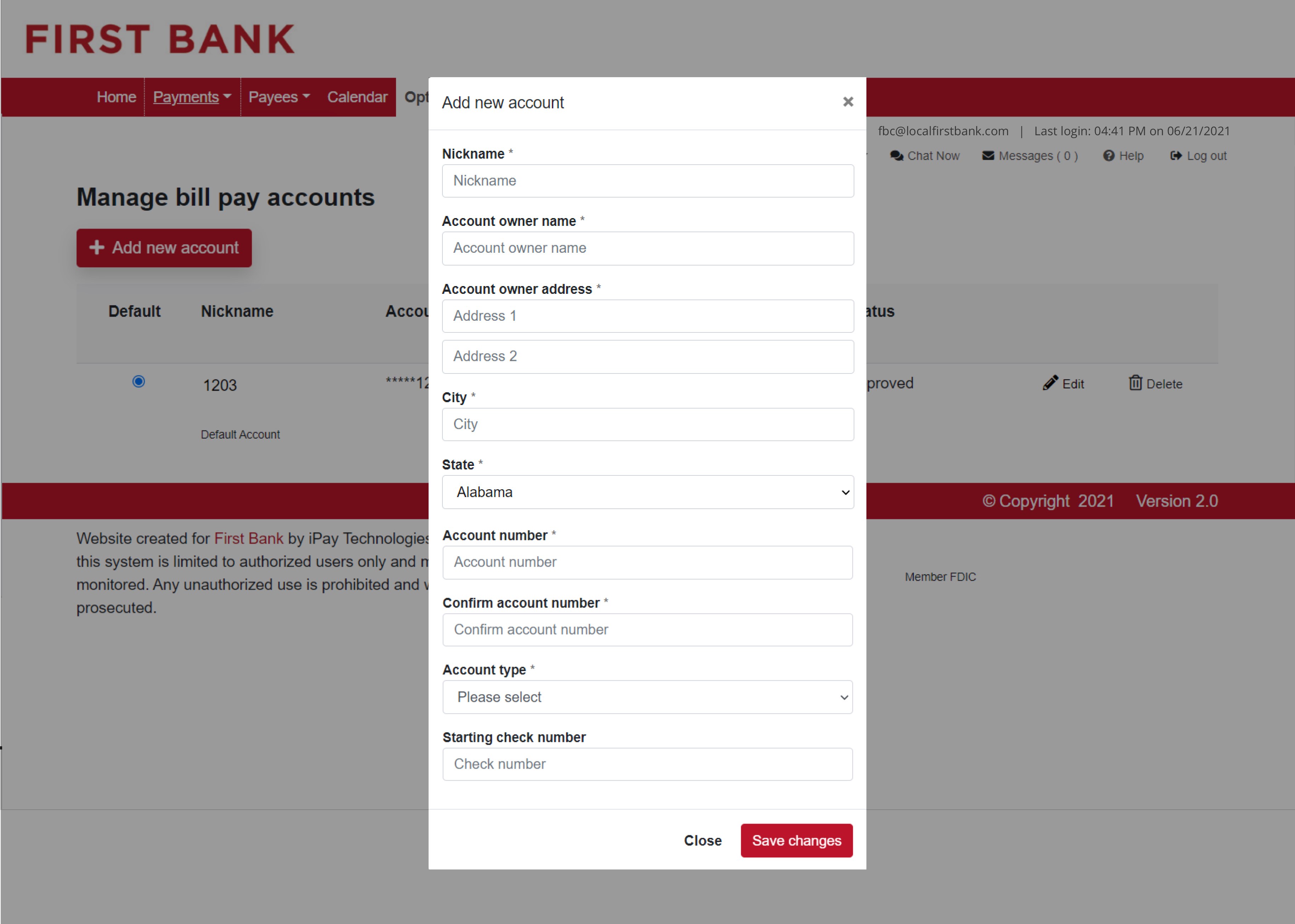This is a detailed view of a FirstBank webpage. The interface is dominated by a grayed-out background featuring the FirstBank logo prominently in the upper left-hand corner. A red navigation bar spans horizontally across the top of the screen with options labeled as "Home," "Payments," "Payees," and "Calendar," each accompanied by a down arrow for additional selections.

On the left side of the page, there's a sidebar displaying the user's last login time, recorded as 04:41 PM on June 21, 2021. This sidebar also includes clickable options for "Chat Now," "Messages," "Help," and "Logout."

A white rectangular pop-up window partially obscures the main page content. The pop-up is titled "Add New Account," with a dismiss button (X) located at its upper-right corner. The form within the pop-up includes fields for "Nickname," "Account Owner's Name," "Account Owner Address" (divided into "Address 1" and "Address 2"), "City," and "State" which defaults to Alabama, with a down arrow for selecting other states. Further fields include "Account Number," marked with an asterisk to denote it as required, and a "Confirmation Number" field, also marked with an asterisk.